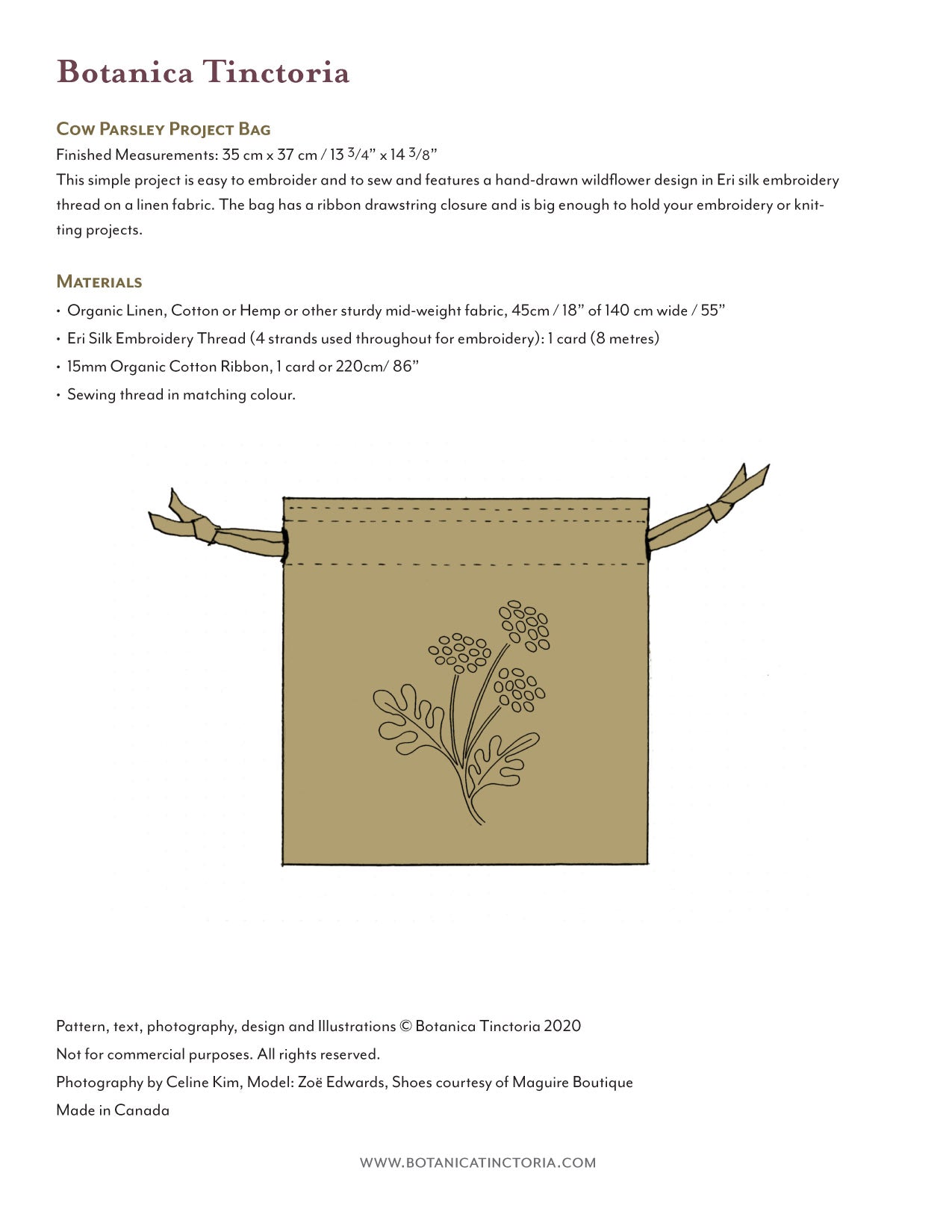The image showcases a page from a book, document, or blog post detailing the Botanica Tinctoria Cow Parsley Project Bag. The finished measurements of the bag are 35 centimeters by 37 centimeters (approximately 13.75 inches by 14.375 inches). This simple, easy-to-embroider and sew project features a hand-drawn wildflower design crafted with airy silk embroidery thread on organic linen fabric. The bag, ideal for holding embroidery or knitting projects, has a ribbon drawstring closure.

Materials listed include:
- Organic linen, cotton, hemp, or other sturdy mid-weight fabric (45 centimeters/18 inches of fabric width 140 centimeters/55 inches)
- Airy silk embroidery thread (four strands used throughout, one card of eight meters)
- Organic cotton ribbon (15 millimeters wide, one card of 220 centimeters/86 inches)
- Matching sewing thread

The visual element includes an illustration of a square bag in an olive drab green color, with a wildflower design adorning the center, and a ribbon drawstring on the sides. The pattern, text, photography, design, and illustrations are credited to Botanica Tinctoria, with 2020 copyright notices indicating no commercial use allowed. The photography is by Celine Kim, featuring model Zoe Edwards, and shoes courtesy of Maguire Boutique. The detailed instructions and imagery provide clear guidance on creating this stylish and practical project bag. For more information, visit www.botanicatinctoria.com.